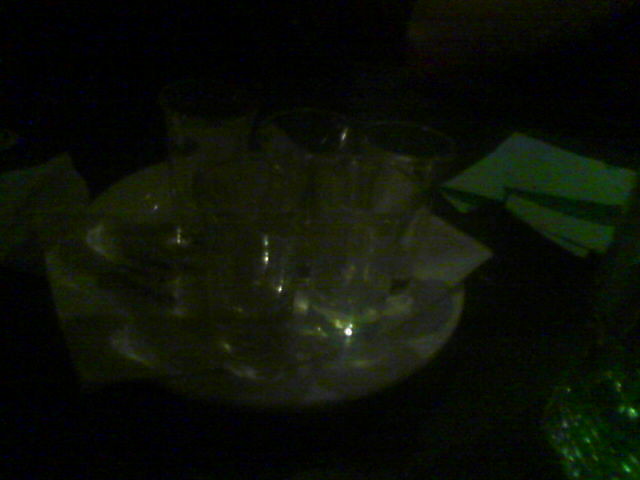The photograph is a dimly lit and out-of-focus image taken in a dark room, making the details hard to discern. At the center, there is a glossy, round white plate with a folded napkin or piece of paper placed over it. Arranged atop the plate are several drinking glasses or tall shot glasses, reflecting a small amount of light likely from a camera flash. To the right of the plate, about midway up, lies another folded piece of cloth or napkin with a floral print. In the lower right-hand corner, a green shape is faintly visible. The overall composition suggests everything rests on a table that blends into the dark background.